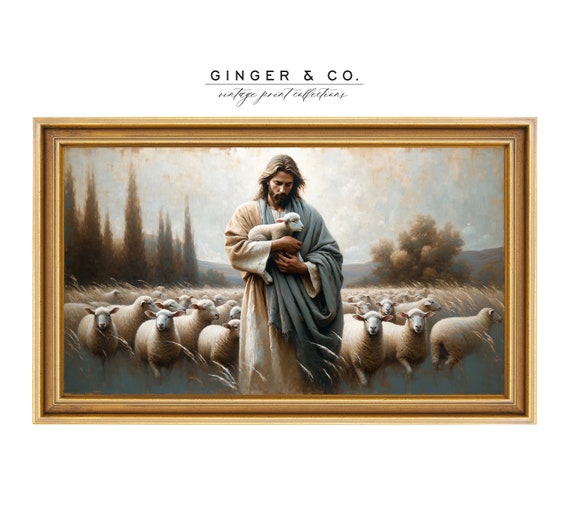This is a framed picture from the Ginger and Co. Vintage Print Collection featuring Jesus in a tranquil pastoral scene. Jesus, with long hair and a beard, is at the forefront of the image, wearing a soiled white robe and a draped pale blue cloth. He lovingly cradles a small lamb in his arms, gazing down at it with a serene expression. Surrounding Jesus is a large flock of sheep standing on a grassy field, with some taller strands of grass at his feet. The natural backdrop includes a mix of tall, thin pine trees on the left and fuller, rounder trees on the right, against a backdrop of mountains and a sky adorned with clouds and subtle golden hues. The frame of the picture is goldish brown, adding an antique quality to the muted color palette of the scene.